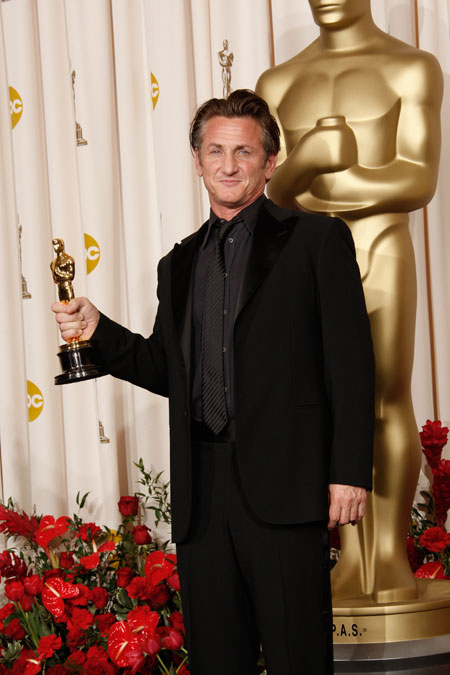In the image, a man is seen standing in front of a cream-colored curtain adorned with numerous circles that have "ABC" printed on them. He is dressed in a black suit, black shirt, and black tie, with his dark hair slicked back and slightly graying at the temples, parted somewhat in the middle. The man is smiling and holding an Emmy award in his right hand, which is positioned with his elbow slightly more than 90 degrees bent. The Emmy statue is gold and stands approximately trophy-sized. Behind the man, the curtain displays images of the Emmy statue, and there is a larger, partially visible gold Emmy statue in the background. Surrounding both the man and the statues are red flowers with green stems, adding a splash of color to the scene.